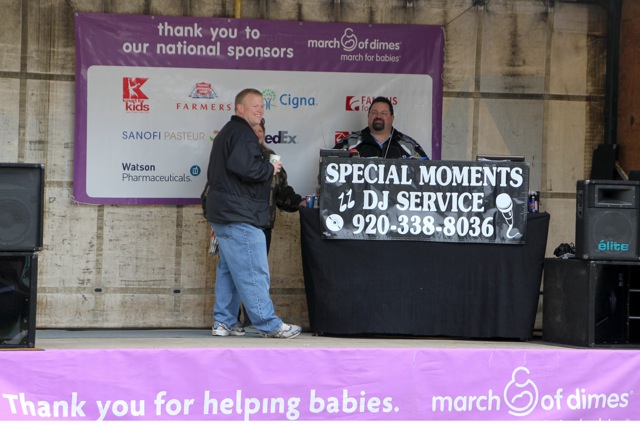The image depicts a rectangular photograph of a stage set up for a March of Dimes fundraiser event, specifically the "March for Babies". The backdrop of the stage is made of white concrete blocks and is adorned with a large purple banner that reads, "Thank you to our national sponsors, March of Dimes, March for Babies." The banner lists various sponsors, including Santa Fe, Cigna, FedEx, and Watson Pharmaceuticals.

On the stage, there is a prominent DJ booth with a black banner on the front that says "Special Moments DJ Service" followed by a phone number, "920-338-8036", in white text. The DJ, a large gentleman with a dark goatee, is wearing a bowling shirt or a black jacket over a shirt, and is positioned behind a black record-playing podium. The DJ is flanked by speakers on both sides: one set on the left and another stack on the right.

To the left of the DJ, two people are visible. One man, appearing to be about 25 to 30 years old with very short hair and wearing a black coat, is smiling and holding a white coffee cup. He is mostly blocking the view of a woman standing next to him, who is only partially visible, identifiable by her ski cap and coat.

The overall atmosphere suggests a cheerful celebration, with the individuals on stage engaging with an unseen crowd in front of them. The detailed arrangements and signage emphasize the collaborative effort of various sponsors in supporting the event aimed at assisting babies through the March of Dimes initiative.